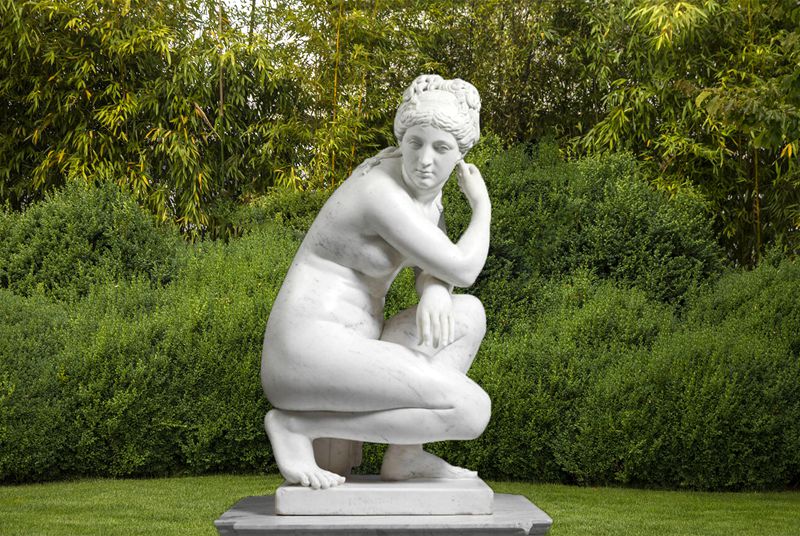The photograph captures a detailed scene featuring a white statue of a woman positioned in an outdoor setting. The statue, which depicts a nude woman with curly hair tied up, is crouching with her right thigh parallel to the ground and her left knee raised. Her face has a stoic and serious demeanor, turned to face the front, offering a side view of her body. The statue is set against a vibrant green backdrop of lush grass, thriving green plants, and tall trees with leaves that appear healthy and radiant under the bright, golden sunlight streaming from above. The entire scene is photographed in a landscape orientation.